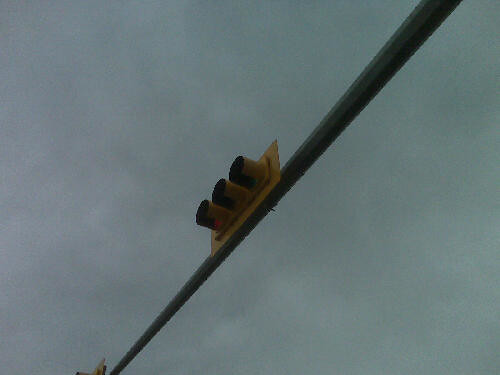This captivating photograph, taken during an overcast day, reveals a unique perspective of a stoplight from below. The image features a long, gray metal arm extending diagonally from the upper right corner to the bottom left, supporting the stoplight. In the bottom left corner, a hint of the yellow border of the signal is visible. The main focus, the stoplight, is seen in its entirety at an angle in the center of the frame. The lights are arranged vertically, with the red light at the top, the yellow light in the middle, and the green light at the bottom. The red light is currently illuminated, indicating that traffic is halted. The image has a slightly dark and grainy texture, adding to the somber mood of the overcast sky.